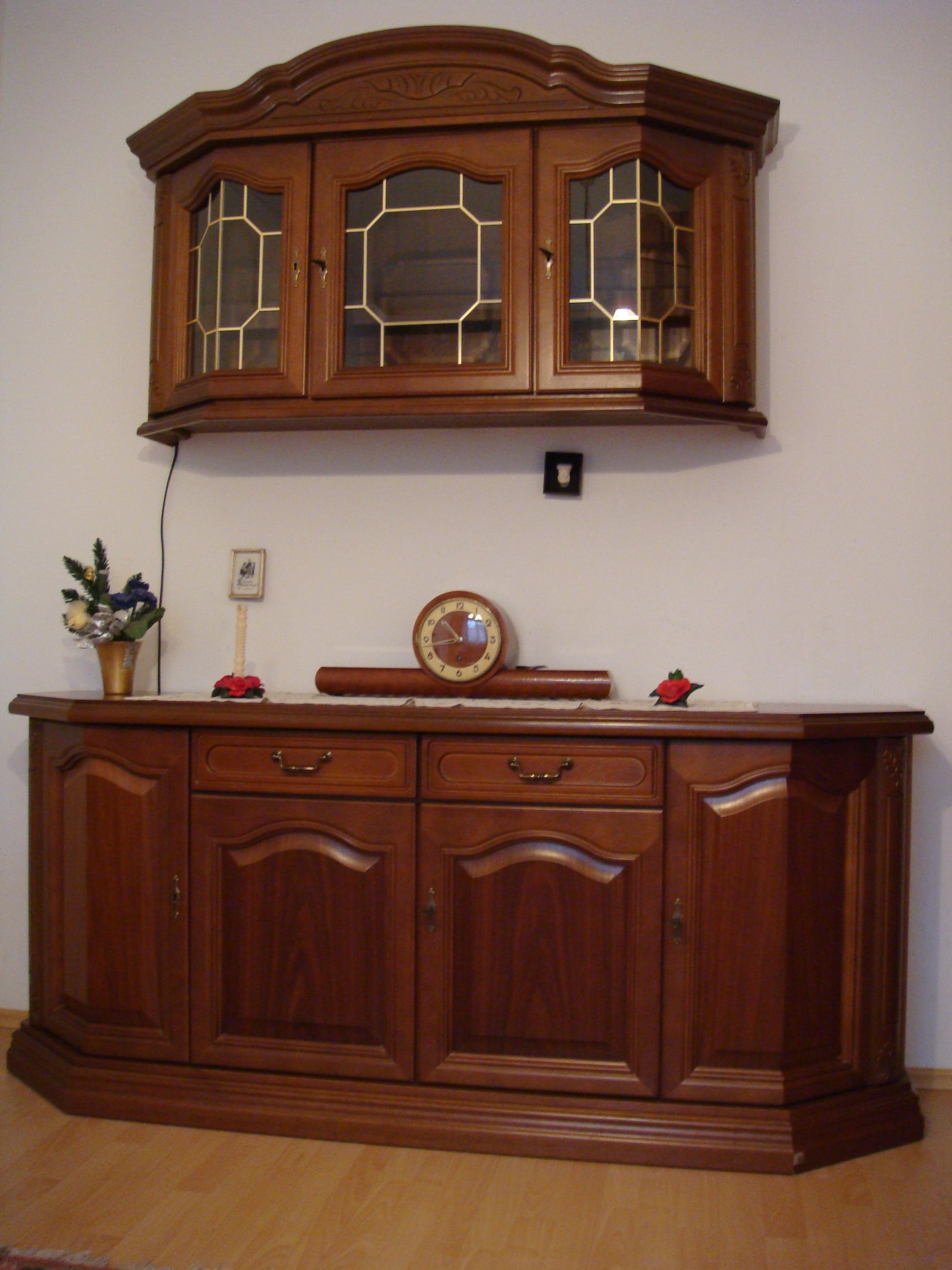This image is a detailed color photograph of a tastefully decorated kitchen scene. At the bottom of the image, there is a medium to dark brown wooden cabinet or credenza with two drawers at the top and two cabinet doors below, sitting on a brown tile floor. On top of the credenza, from left to right, there is a gold pot with plants, a red rose in a small vase, a brown table clock with a horizontal stand in the center, and another red flower with a decorative candle. Above the credenza, mounted on a white wall, is a glass-fronted wooden cabinet with a curved top and a flat bottom. The cabinet has three windows outlined in gold with geometric shapes. Just below the glass-fronted cabinet, there is a power outlet on the wall. This meticulously arranged setting combines functional furniture with elegant decor, providing a warm and inviting ambiance.